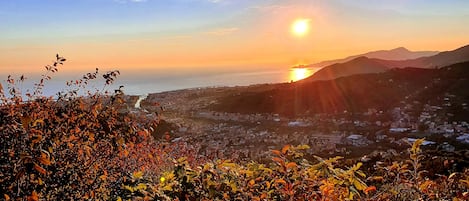This detailed panoramic photo captures a serene outdoor scene likely set on an island. In the immediate foreground, various foliage, including bushes with a mix of green, brown, orange, and white leaves, stretches diagonally from the front left to the bottom right of the image. Beyond the foliage, there is an expanse of land with varying elevation levels that lead the eye towards a body of water. This water, a deep blue, reflects the bright orange sun that hangs in the sky on the right side of the image. The sky above transitions from the blue of day to the soft orange hues of sunset, with wispy white clouds scattered throughout. Towards the background, a small town with several buildings, possibly markets and houses, can be seen. Further still, there are more distant structures and the silhouette of mountains. A trail winds through the scene, adding depth and leading towards the peaceful horizon, which is expansive and devoid of human activity, evoking a sense of tranquility and calm.